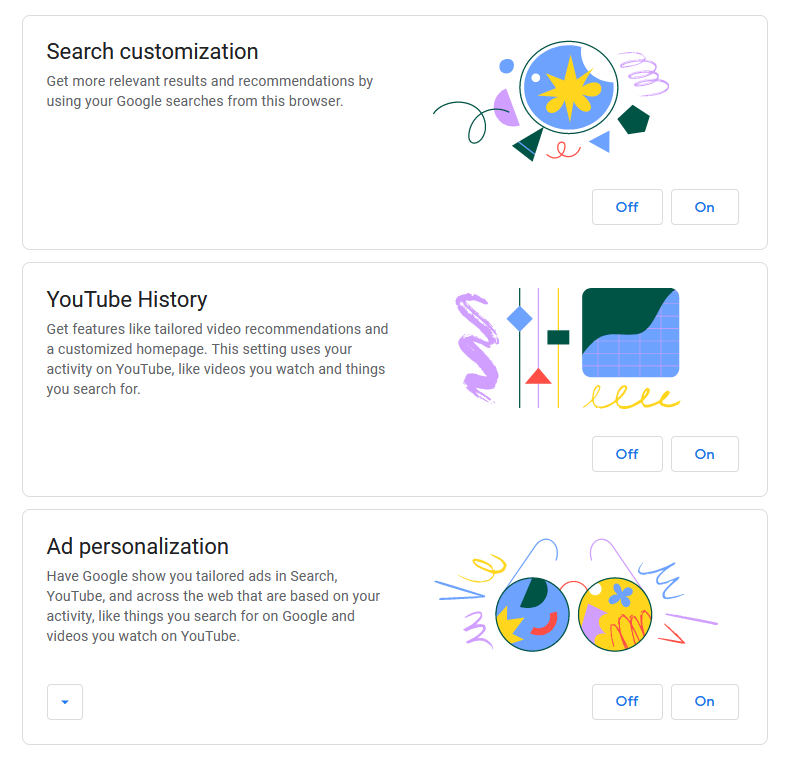The image is divided into three rectangular sections of information, each detailing ways to personalize your Google experience. 

**Section 1: Search Customization**
This section explains how to get more relevant results and recommendations through Google Search based on your activity within the browser.

**Section 2: YouTube History**
This section highlights features like personalized video recommendations and a customized homepage on YouTube. It mentions that tailored content is created using your activity on YouTube, such as the videos you watch and the things you search for.

**Section 3: Ad Personalization**
This section discusses how Google can provide tailored ads in Search and YouTube, as well as across the web, based on your activities like Google searches and YouTube video views.

Each section also features a toggle switch on the side, indicating that these settings can be turned on or off as desired.